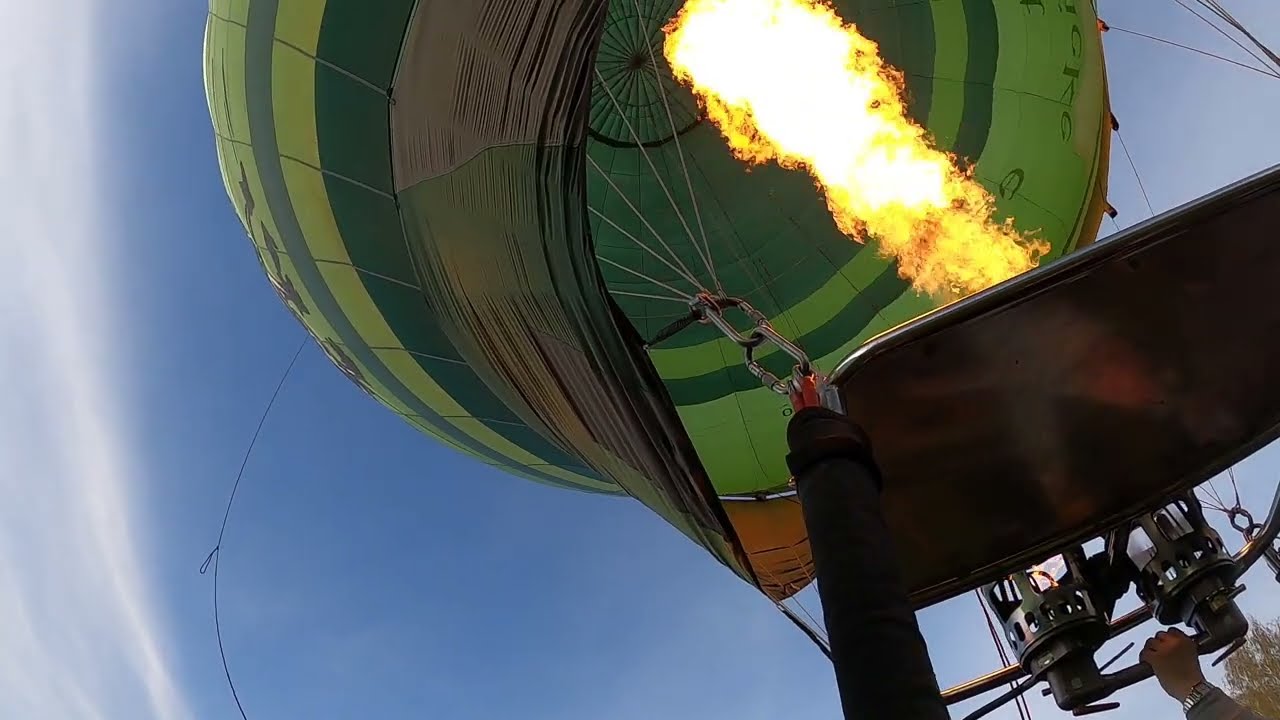The photograph captures a dynamic moment from the perspective of within or just outside the basket of a hot air balloon. The focus is on the large, intense flame being released by the operator, whose hand—adorned with a watch—pulls down the lever to ignite the torch. The fire, a huge and vivid burst, climbs up into the balloon to heat it, with flames extending several feet skyward. The balloon itself features a design primarily in yellow-green and dark green stripes, with a hint of gray at its bottom edge. A subtle, indistinguishable design marks the center of the balloon. Above, the sky is a brilliant blue, accented with a few wispy clouds. The intricate web of cables and clips securing the balloon to the basket is clearly visible. Below, there is a hint of some small trees in the corner, suggesting that the balloon is either preparing for lift-off or has just begun to ascend. The image effectively conveys the powerful energy and preparation involved in balloon flight.